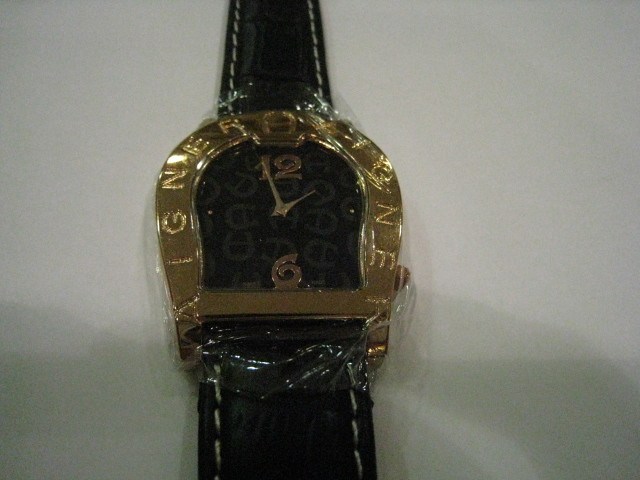This image features a unique wristwatch set against a solid white background, exhibiting subtle shadowing at the bottom likely cast by the person taking the photo. The watch stands out with its thin black leather band, accentuated by delicate white stitching along the edges. The band runs vertically through the image. The watch face is framed by a distinctive gold horseshoe-shaped casing, which includes a horizontal bar at the base of the horseshoe. The watch face itself is black, with the numbers 12 and 6 prominently displayed in gold. The rest of the face features a faint gold pattern that mirrors the horseshoe shape seen in the casing. Additionally, there is some text on the watch, which appears to spell "IGNER" or "INGER," though it is somewhat obscured by a protective plastic wrap.